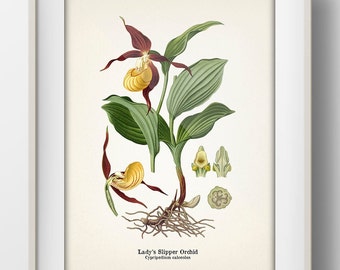This is a framed illustration, resembling a poster, of a Lady Slipper Orchid. The frame of the picture is white, complementing the white background of the image itself. The central focus is an orchid with a distinctive yellow cup-shaped appendage at its center, surrounded by deep reddish-purple, slightly wilting petals. The orchid is attached to a green stem that displays several rich green leaves with detailed linear patterns. The roots of the plant are visible, showcasing a reddish hue. At the bottom of the illustration, the text "Lady Slipper Orchid" is clearly visible, though additional fine print lettering is too small to read.